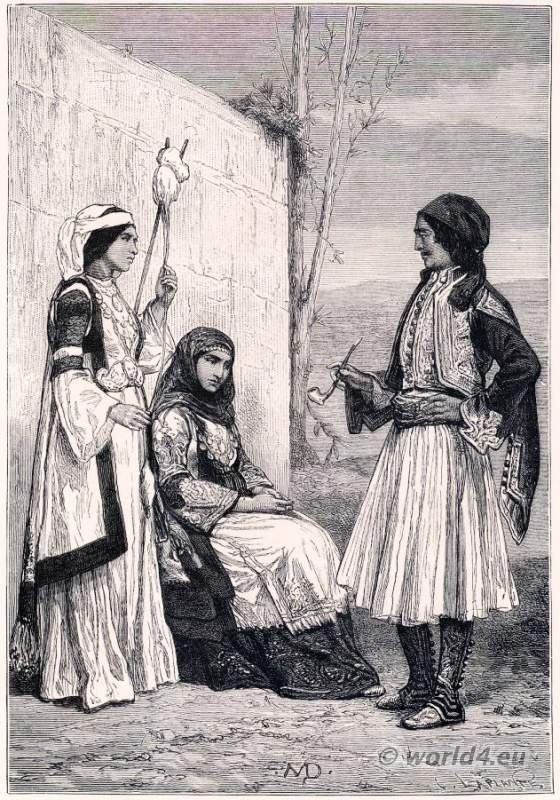This detailed pencil drawing or painting, presented in black and white, captures an outdoor scene where three individuals are positioned against a white stone wall with a barren tree and rolling hills in the background. The image has the annotation "world4.eu" at the bottom.

On the left, a woman stands slightly behind and to the right of another woman who is seated in a chair. The standing woman has her head wrapped in a white headscarf that covers her black hair. She wears a long, ruffled white gown topped with a contrasting black and white overcoat, holding a staff with a cotton-like top in her left hand. The seated woman wears a head covering that conceals her hair but not her face. She’s dressed in a heavily embroidered long-sleeved blouse with an apron over her long skirt, her hands folded neatly on her lap as she gazes downward.

On the right, facing them is a man with a dark mustache, also in profile. He wears a headscarf over long hair, a gold-trimmed overcoat, and a white pleated skirt reaching down to his ankles. His right hand holds a long-necked pipe near his waist while his left hand rests on his hip. The intricate details of their garments and their composed poses contribute to the historic and cultural richness depicted in this illustration.